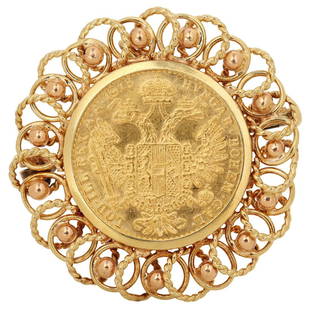The image features a detailed, circular pendant or medallion, resembling an antique gold coin at its center. This central portion appears to bear a crest, with a two-headed bird whose wings are outstretched. A crown is positioned between the bird's heads, which face in opposite directions. Surrounding the central coin is textured, yet hard-to-read writing, which blends into the gold background.

Encircling the coin are intricate, overlapping rings designed in a two-toned gold pattern—some sections of bright yellow gold and others of a more subdued rose gold. Small, pinkish circles are embedded within alternating rings, contributing to the elaborate filigree design. The outer rings are less shiny compared to the central medallion, giving the entire piece a decorative look, akin to a keepsake or an ornamental wall hanging.